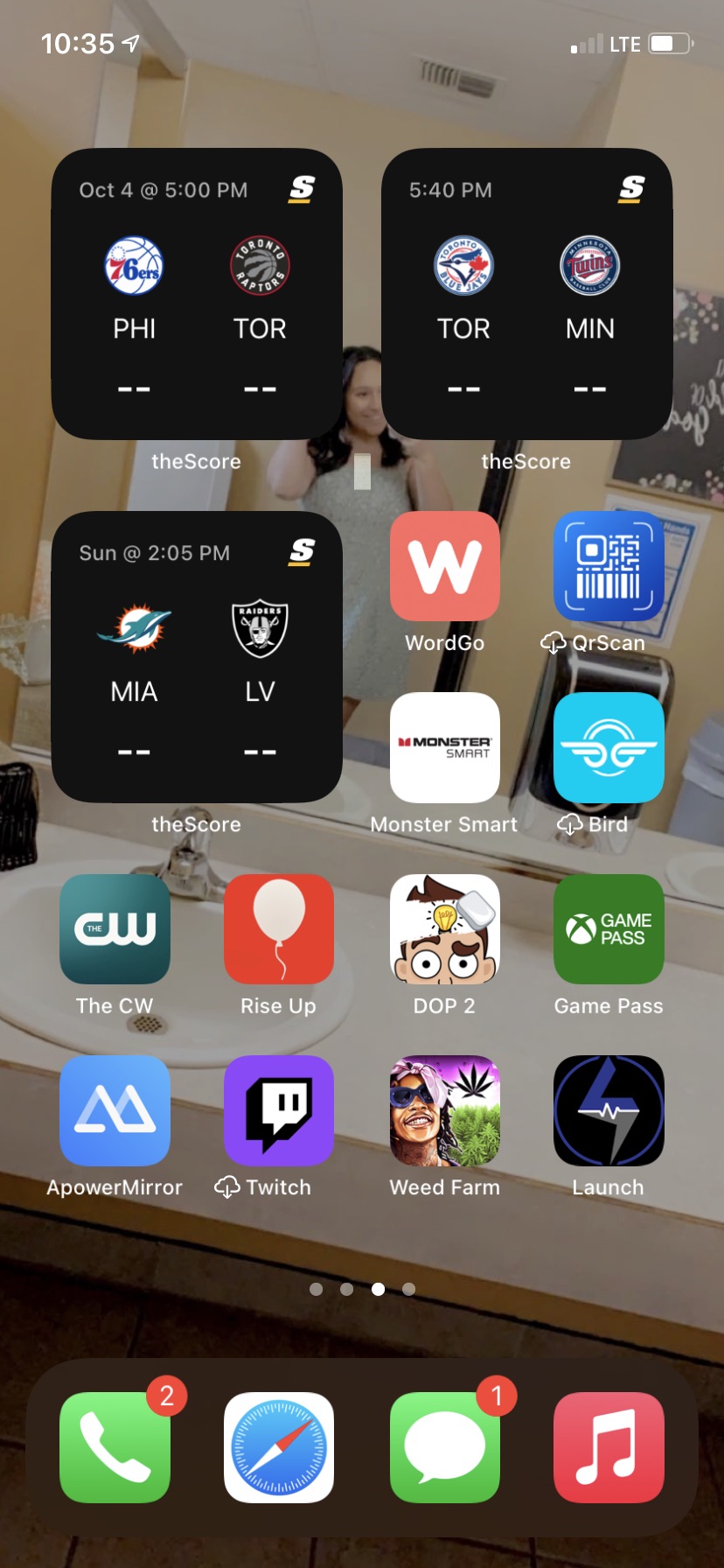The image depicts the home screen of a smartphone. The wallpaper in the background features a person taking a selfie in a bathroom. The time displayed at the top of the screen is 10:35, and the phone appears to be using mobile data rather than Wi-Fi. The date, October 4th, is shown, along with reminders for two sports events: "Phillies vs. Toronto" at 5:00 PM and "Toronto vs. Minnesota" at 5:40 PM.

Numerous app icons are displayed on the home screen. Some of the prominent apps include:

- **Word Go**
- **Bird**
- **Monster Smart**
- **The CW**
- **Rise Up**
- **Game Pass**
- **Power Mirror**
- **Twitch**
- **Weed Farm**
- **Launch**

Additionally, there is a phone icon indicating two missed calls, a maps icon, and a messaging icon showing one unread message. A music app icon and an app named "DOP2" are also visible, along with a QR scan option.

This detailed and descriptive observation captures the essence of the phone's home screen and the various applications and notifications displayed on it.